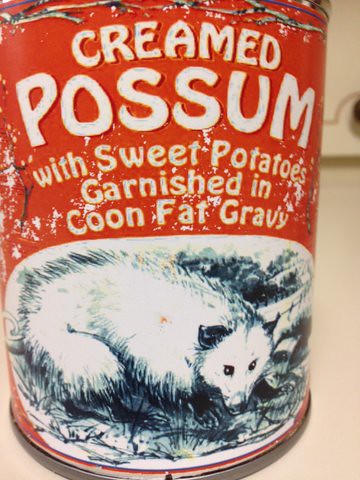The image is of a vintage, red aluminum can labeled "Creamed Possum with Sweet Potatoes Garnished in Coon Fat Gravy." The text is in bold white letters on a red background. The can, which appears to be slightly dented and shows some gray and white areas around the top, features a detailed black and white sketch of a possum on the bottom half. The possum is depicted sitting on grass amidst foliage and shrubs, with distinctive black ears, black eyes, a long nose, and long fur. This elaborate and somewhat peculiar label gives the impression it could be a novelty or joke item.